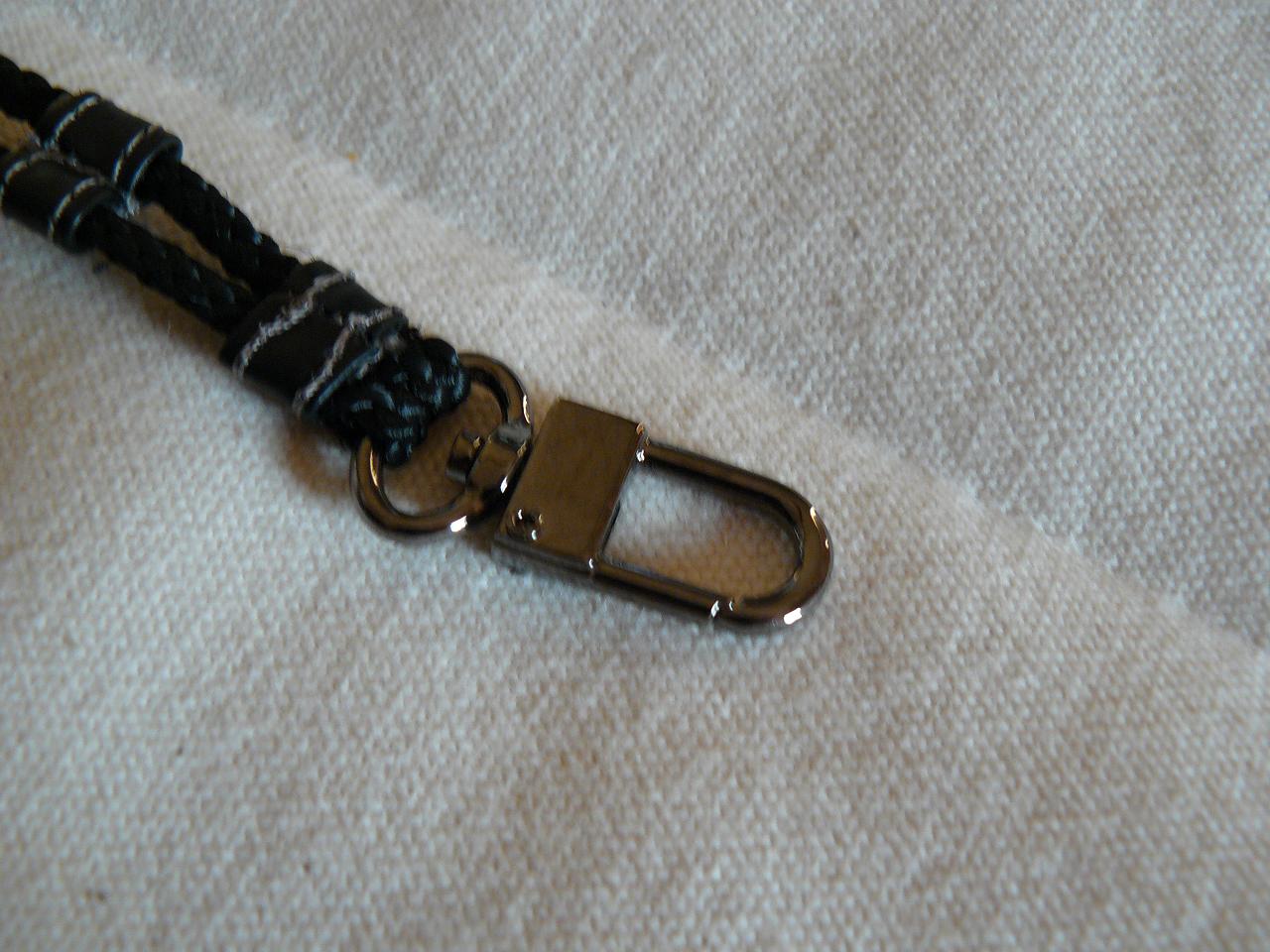The image depicts the detailed end of a chain or necklace made from string. Attached to this string are four small, dark blue bands, with two bands positioned near the top and stitched together with gray thread closer toward the base. These bands appear to be made of leather or faux leather. The chain ends in a metal ring, which houses a swivel attachment featuring a metallic loop reminiscent of a master lock, all made of possibly stainless steel. The entire setup is laid on a white, thickly textured fabric, similar to a canvas or thick paper towel, with the chain and swivel angled towards the lower right. The photo is highly magnified, revealing intricate details of both the chain and the fabric's stitching.